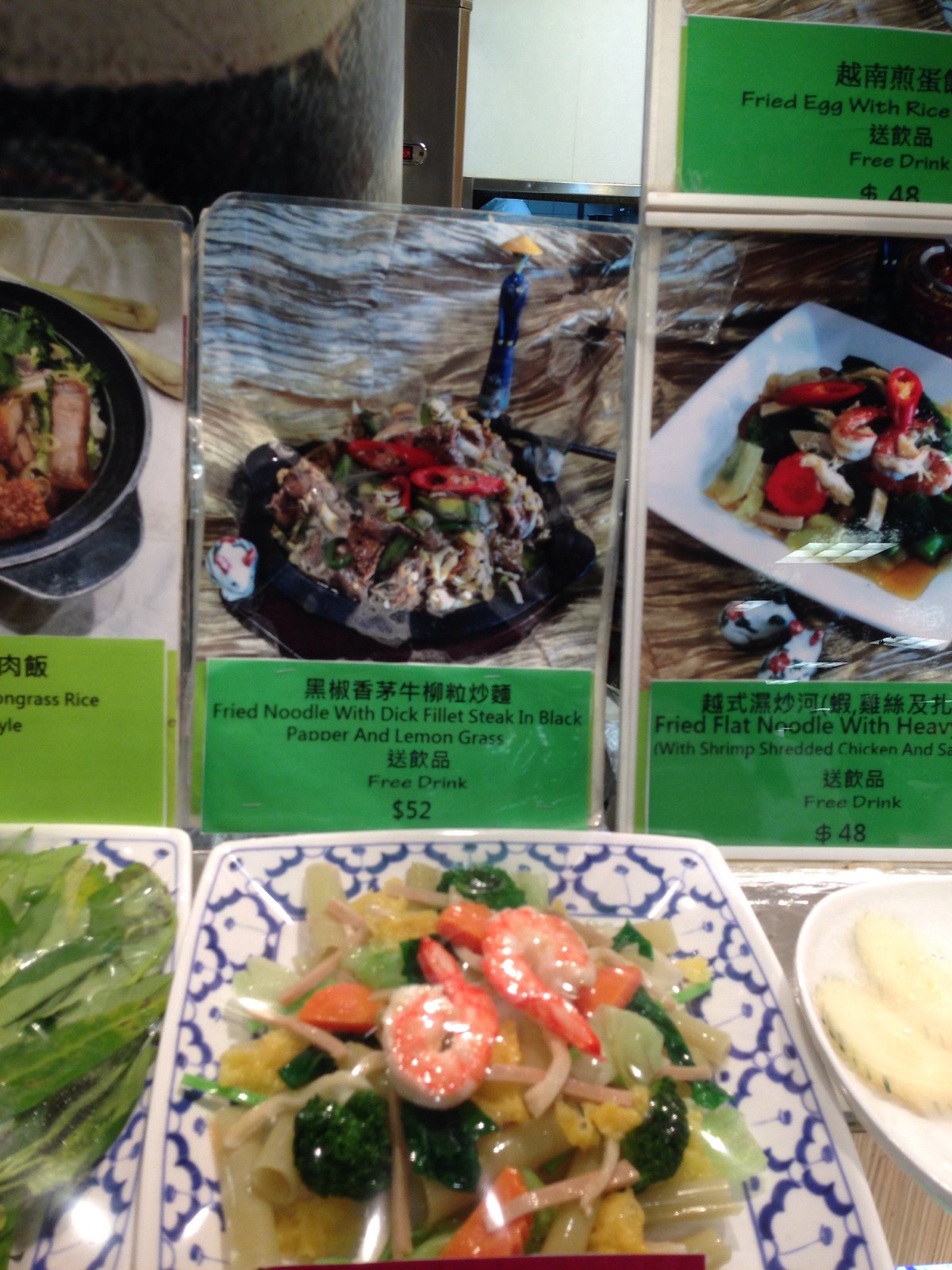The photograph displays an assortment of neatly arranged Asian dishes, with an emphasis on Chinese cuisine. Dominating the bottom portion of the image is a white plate adorned with intricate blue floral patterns, piled high with vibrant vegetables, including bean sprouts and broccoli, alongside shiny, delectable shrimp that catch the ceiling's light. Above and to the side of this primary plate, various other dishes are visible. To the left, one can spot leafy greens, and to the right, something resembling a banana on a white plate. 

Central to the image is a picture of a black dish containing red peppers and meat, labeled “Fried Noodle with Steak Finage: Steak in Black Pepper and Lemongrass, Free Drink, $52.” Adjacent to it, partially cut off, is another description indicating “Fried Egg with Rice and Free Drink, $48.” A third dish, partly obscured, lists “Fried Flat Noodle with Heavy,” mentioning shrimp, shredded chicken, and another ingredient that is cut off.

The background features more arranged saran-wrapped dishes and corresponding photos with descriptions and prices, providing a visual menu that captures the variety and richness of the offerings. On the very right, there appears to be a door with a glass panel, enhancing the setting's authenticity. The photograph is a vibrant display of Asian culinary delights, meticulously described and invitingly presented.